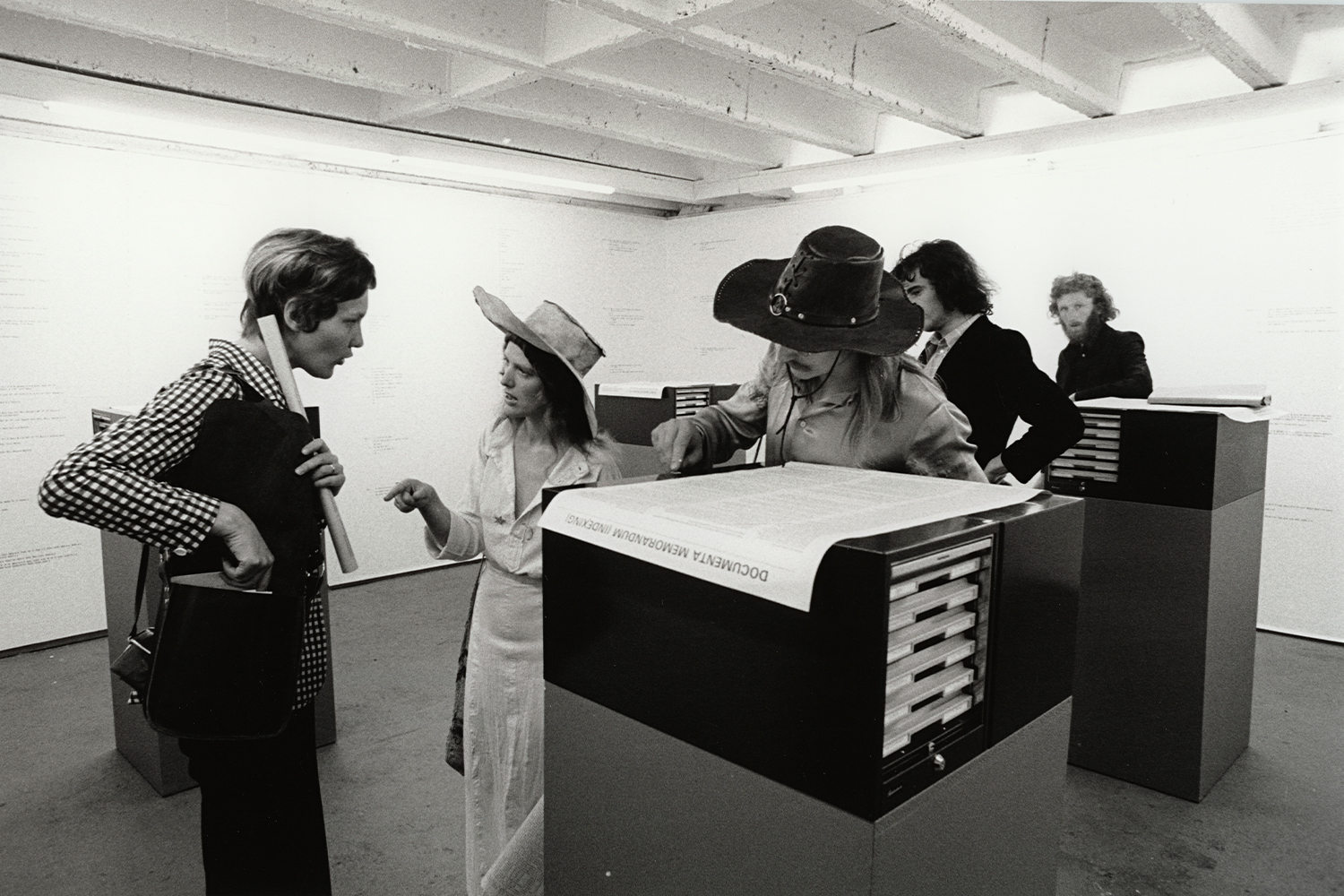This black and white photo captures five people standing in what appears to be a small room, potentially an art gallery, with stark white walls that emphasize the figures within. Central to the image is a man donning a cowboy hat and a beard, intent on something atop a black chest-high pillar, which seems to be adorned with a newspaper or a large piece of paper. Surrounding him are four additional figures: to his left, a woman in a white dress and sun hat gestures while conversing with another woman. This second woman is clad in a checkered blazer, holding a rolled-up paper in one hand and a large black satchel on her side. Behind the central man, two more men, both dressed in dark clothing, stand in the background, adding layers of intrigue to the scene. The room's minimalist setup consists of four black pillars or table-like structures, each topped with paperwork, providing a focal point for the individuals' interactions.